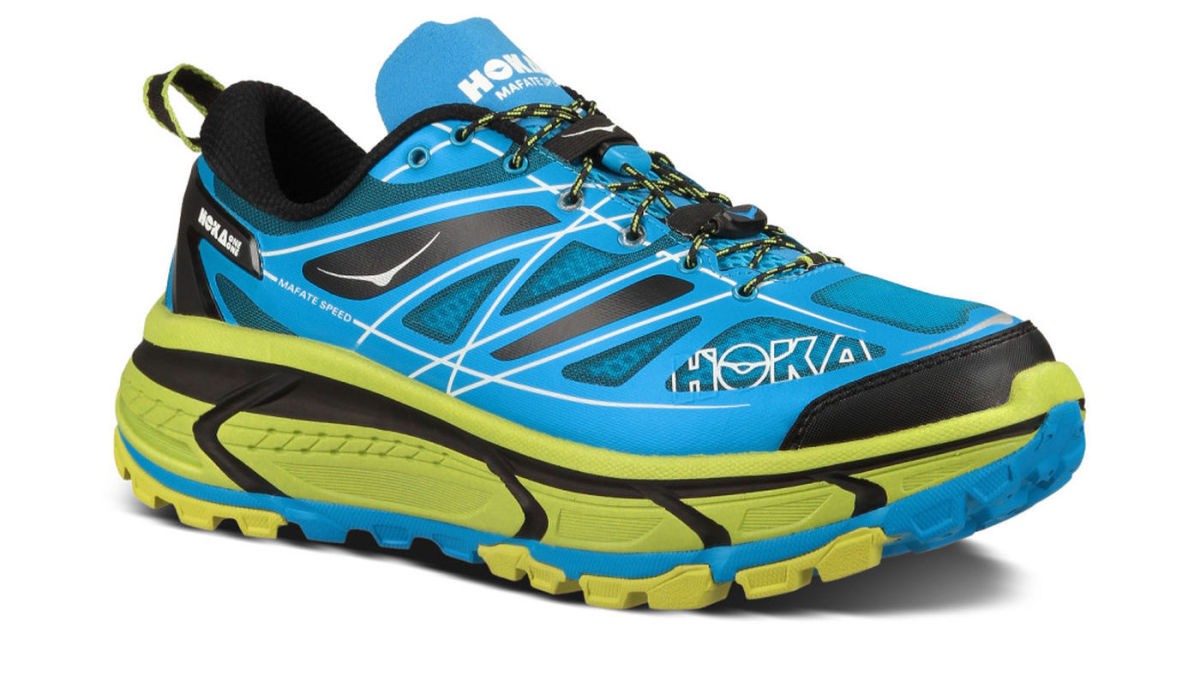This is a vibrant, modern Hoka gym sneaker primarily featuring a light robin's egg blue color. The toe is on the right and the back is on the left. The sneaker is detailed with thin white lines running throughout the top, creating sections adorned with black and blue geometric shapes. Prominent white block letters spelling "HOKA" are visible on the side, tongue, and back of the shoe. The sneaker is accented with a black trim around the back. The laces are a contrasting combination of black and yellow. The sole of the shoe is an eye-catching mix of yellow with blue and black trim, and a distinctive green strip runs along the side and back. The rubber bottom is lime green, enhancing the clean, sleek look of the shoe.